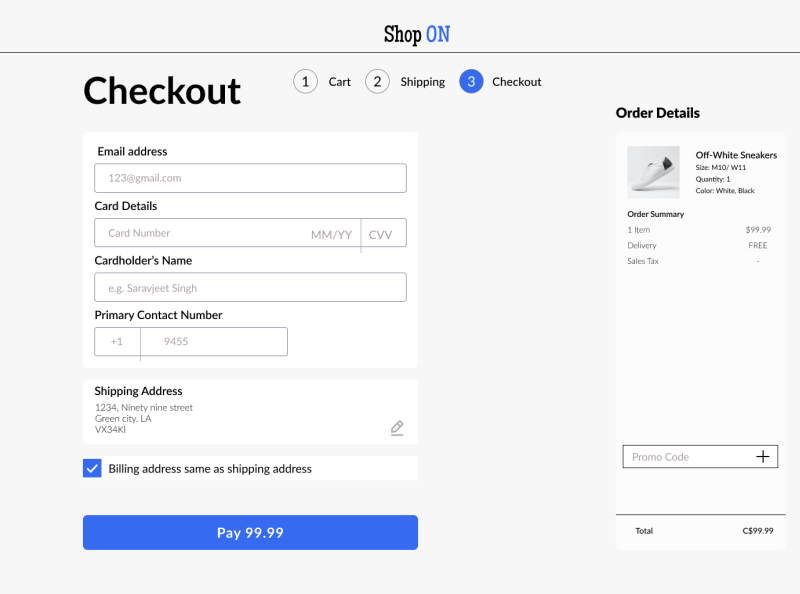**Detailed Caption for Website Checkout Page Image:**

The image displays the top section of an e-commerce website's checkout page, focusing on the specified phases of the checkout process. At the top center, the word "Shop" is prominently displayed, followed by a progression bar labeled "1 Cart," "2 Shipping," and "3 Checkout," with "3 Checkout" highlighted in blue, indicating the current stage. 

Below this, there is an empty field for the email address. Underneath the email section, there are fields for the cart details, which are currently blank, including "Card Holder Name" and "Primary Contact Number." The "Shipping Address" is filled in with "1234 99th Street, Green City, Louisiana, BX34KL." 

The "Billing Address" is shown as "Same as Shipping Address" with a blue checkmark beside it, confirming the selection. A prominent blue rectangular box at the bottom contains the label "Pay $99.99."

On the top right section of the page, "Order Details" are mentioned, featuring a small thumbnail image of an off-white sneaker. The sneaker is listed as "Off-White Sneaker," size "M10/W11," with a quantity of one in the color combination "White/Black." An "Order Summary" follows, detailing one item costing $99.99, with free delivery and blank sales tax. 

At the bottom of this summary, there is a section labeled "Promo Code" with a plus sign next to it, indicating the option to apply a code. The total amount is highlighted as $99.99.